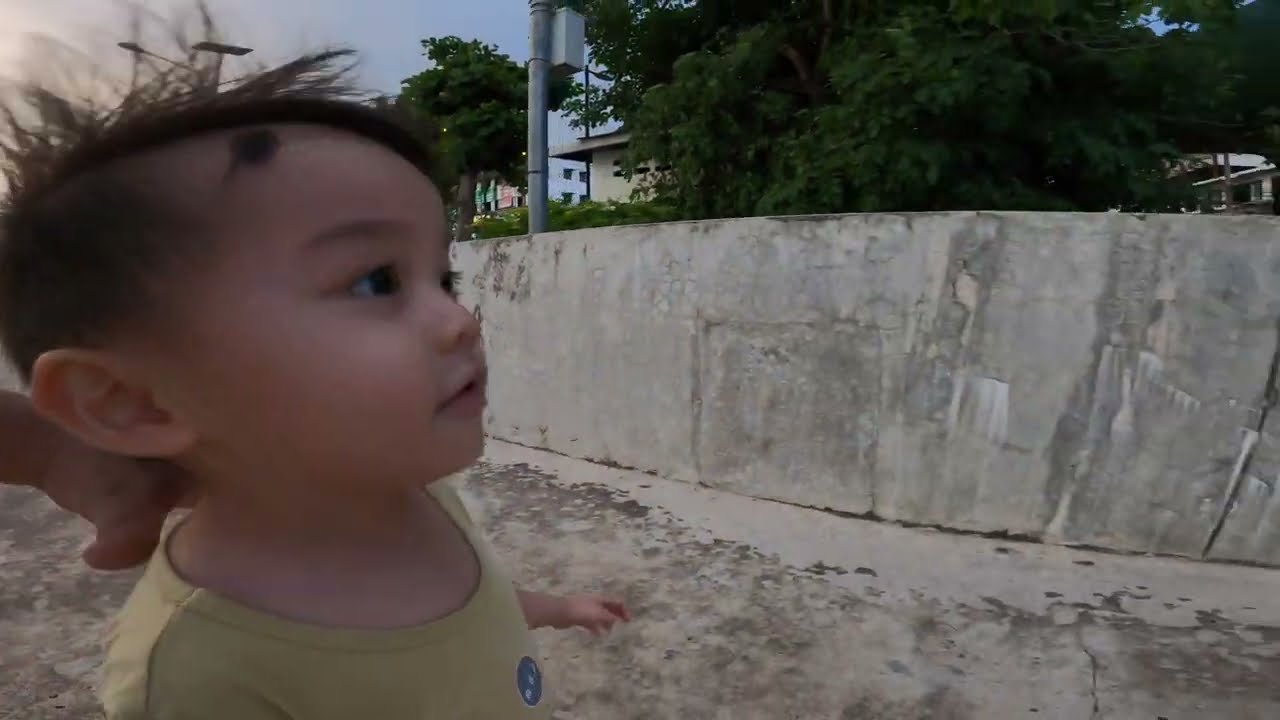The photograph captures a close-up of a little boy, who appears to be of Asian descent, with messy black hair that has a few thin patches revealing a prominent mole on his scalp. The boy, likely under two years old, is positioned on the left side of the frame. He is looking to the right with his mouth slightly open, offering a side profile view. He is dressed in a short-sleeved shirt, predominantly yellow or greenish-yellow with a small blue circle on the chest area. The boy's left hand is outstretched in front of him, and another hand, likely of an adult, is visible behind his neck, suggesting someone is guiding or supporting him.

The background consists of a grey cement wall and a similarly colored concrete ground, which shows signs of dirt and black marks, indicating it's quite worn. Rising above the wall, there's a large green tree occupying much of the upper part of the view. To the left of the tree, portions of white buildings are partially visible through the foliage, indicating an urban environment beyond the immediate setting. The detailed composition creates a vivid portrayal of the boy in his surroundings.